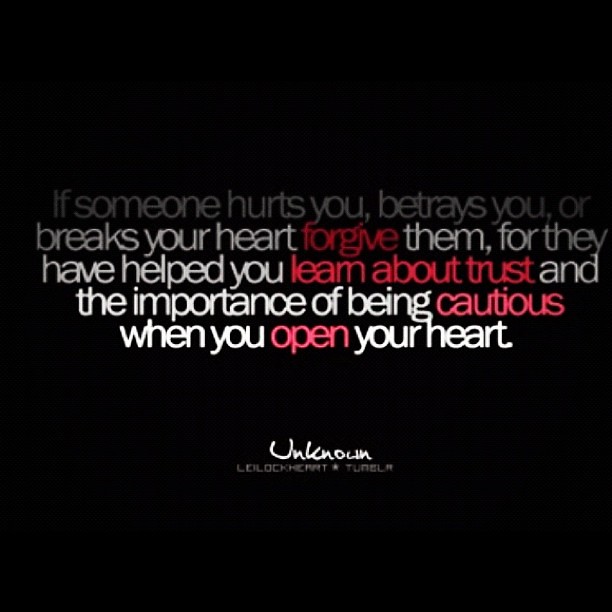The image is a square poster with an inspirational quote on a black background. The text at the top is somewhat faded and becomes more pronounced towards the bottom. The quote reads: "If someone hurts you, betrays you, or breaks your heart, forgive them, for they have helped you learn about trust and the importance of being cautious when you open your heart." Key words such as "forgive," "learn about trust," "cautious," and "open" are highlighted in deep red. The quote is attributed to an "Unknown" author, and there's additional smaller, blurry text at the very bottom, which appears to say "Lyle Lockhart" or something similar.